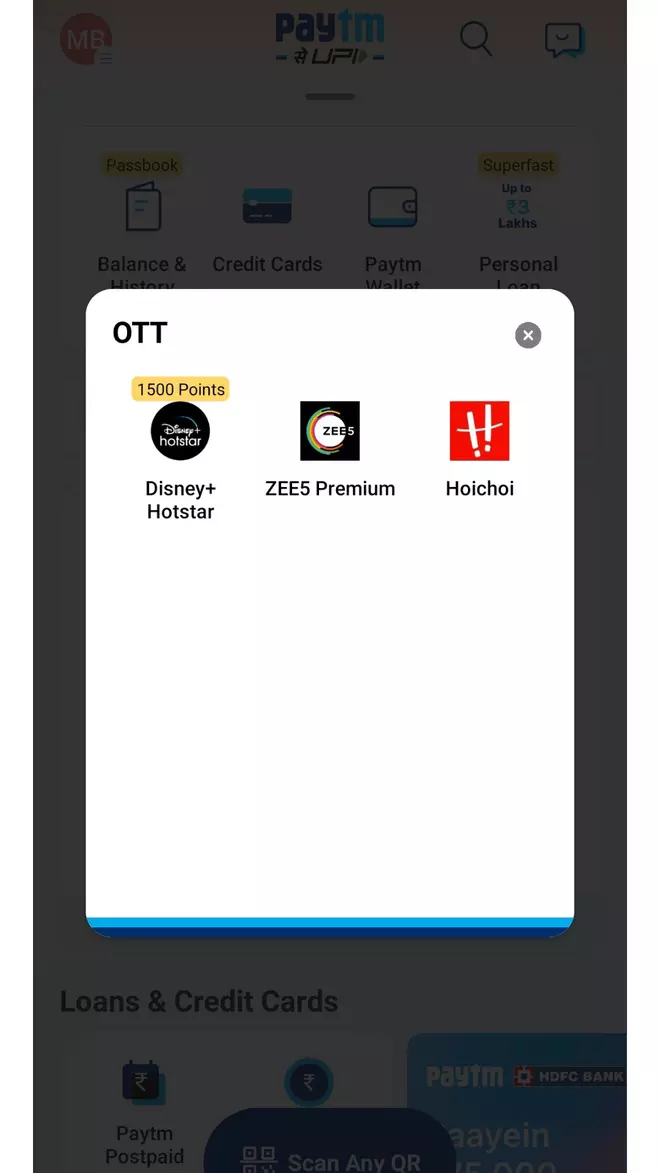The image is a screen capture displaying an overlay on top of another screen, with the background screen grayed out. The background features a predominantly white interface with several colored icons. At the top-left corner, a blue circle with the letters "PAYTM" is visible. Moving across the background screen, other elements include a magnifying glass icon, a square icon, and various functional icons labeled with descriptions.

These icons include:
- A "Balance and History" section represented by a small ledger symbol.
- A "Credit Cards" icon featuring a blue credit card.
- A "Payment Wallet" icon depicted with a white wallet having a blue stripe.
- Additional unspecified icons.

Towards the bottom-left of the background, there is a section labeled "Loans and Credit Cards," beside a blue box suggesting the option to scan a QR code for payments.

Overlapping this background interface is a dominant white box labeled "OTT" in black text. This box includes three icons related to streaming services:
1. **Disney Hotstar**: A navy round circle with white text, stating "1,500 points" above it.
2. **ZEE 5 Premium**: A black square with a white circle, accented with green and orange hues, featuring the text "ZEE 5" across the circle.
3. **Hoichoi**: A red-orange icon with a white "H" and the text "Hoichoi" spelled out.

In the top-right corner of the white overlay box, there is a grey "X" for closing the overlay, and a thin blue line runs along the bottom edge of the white box.